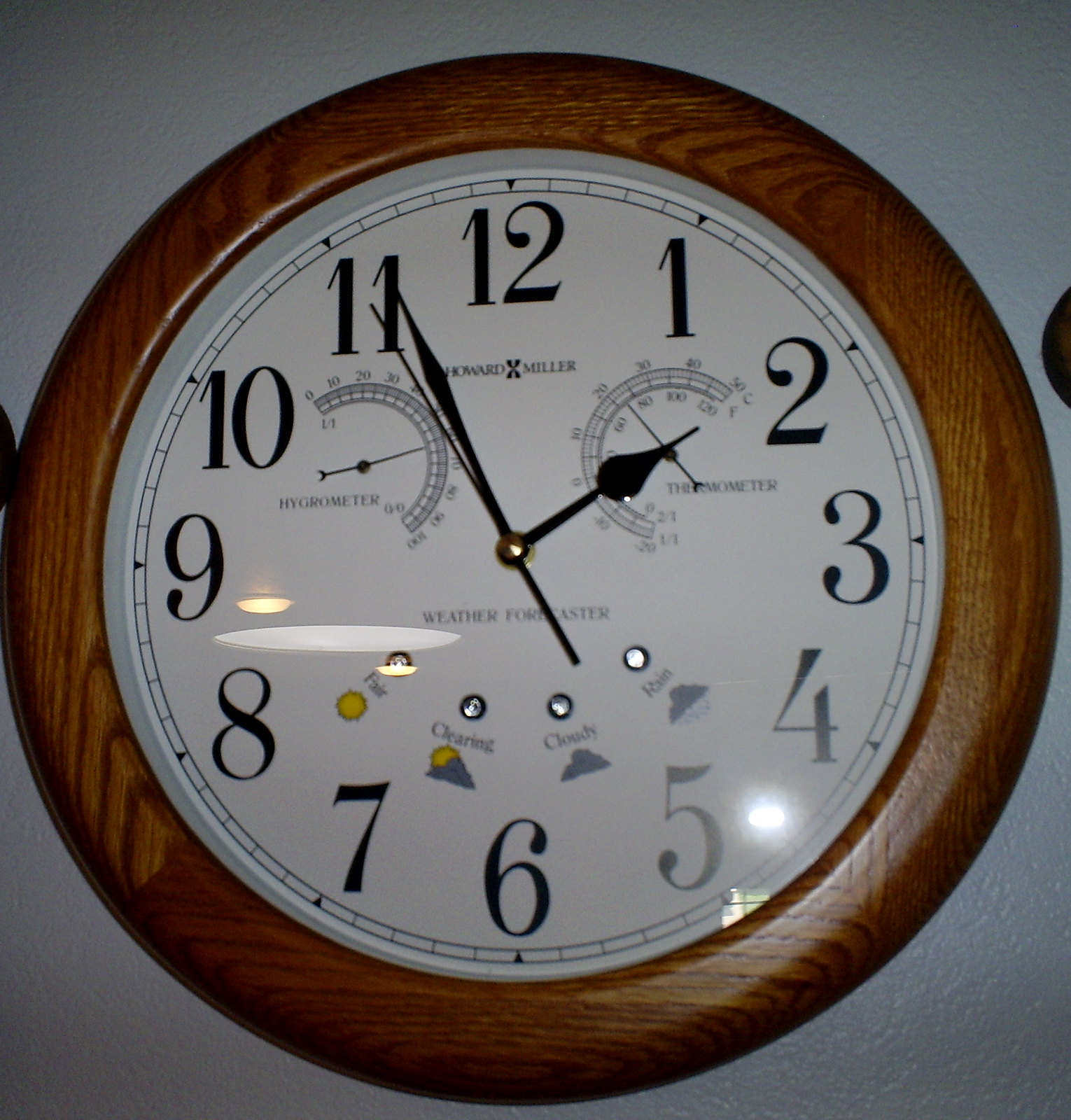This video captures a wooden analog clock mounted on a slightly textured white wall. The clock's circular frame is made of medium-colored, oak-toned wood with visible grain, complementing the clean, white face. Prominent, easy-to-read black numbers encircle the clock, and the hands—featuring a thin second hand, an elongated diamond-shaped minute hand, and a spade-tipped hour hand—indicate 1:55, with the second hand pointing towards 11. Above the center where it states "Weather Forecaster," two smaller dials include a hygrometer to the left of the 10, and a thermometer near the 2, displaying approximately 74°F (23°C). Below this section, a sequence of four dots is methodically positioned with small icons depicting different weather conditions: "Fair" with a sun between the 7 and 8, "Clearing" with a sun emerging from clouds between the 6 and 7, "Cloudy" depicted with clouds between the 5 and 6, and "Rain" showing a cloud with rain between the 4 and 5. The clock, manufactured by Howard Miller, combines traditional timekeeping with practical weather forecasting tools.